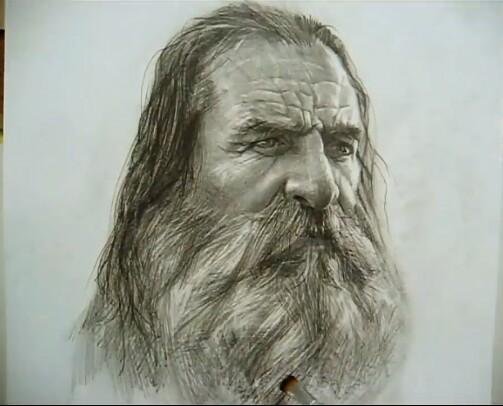This highly detailed, photorealistic black and white drawing, possibly rendered in charcoal or pencil graphite, features the face of an elderly man set against a white background. His long, greasy-looking hair falls back to his shoulders, blending seamlessly into his extensive facial hair. His large, somewhat bushy beard, paired with a thick mustache that covers his upper lip, envelops his entire face. The man’s expressive, piercing eyes are framed by dark, furrowed eyebrows and deep wrinkles, particularly on his forehead, accentuating his intense, squinting gaze. The drawing captures the texture and age lines on his face, emphasizing a sense of wisdom and contemplation.